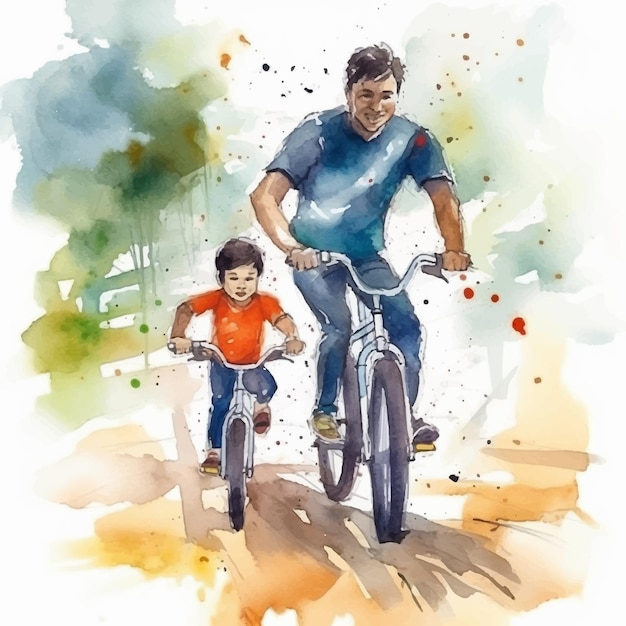The image depicts a vibrant watercolor painting of a father and son riding bicycles towards the viewer. The man, positioned in the center-right, is dressed in a short-sleeved blue shirt and blue jeans. His footwear is somewhat mismatched, with what appears to be a sneaker on his left foot and a possibly open-toed sandal on his right. The young boy, positioned to the man's left, wears an orange (appearing sometimes as red) t-shirt and blue jeans, and rides a smaller bike identical in design to his father's larger one. Both figures have short dark hair and are prominently displayed in the middle of the image. The road beneath them is crafted with shades of brown, orange, and tan, indicative of watercolor's fluid and textured tones. The background features splashes and splotches of blue and green, intermingled with speckles of various colors like orange, gold, black, and green, lending the scene a lively, dynamic feel. The painting captures a moment of shared joy between the father and son, richly embedded in the colorful, abstract surroundings suggestive of a carefree day spent together.